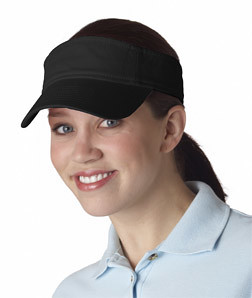The photo is a detailed head shot of a young woman with a distinct yet subtle charm. She has bright blue eyes and is wearing red lipstick that highlights her friendly smile, revealing the top row of her teeth. Her skin is pale and her cheeks have a slight rosiness. She wears a black cap, which is likely a baseball cap with a gray area around the front bill. The cap secures her dark brown or black hair, which is pulled back into a ponytail, keeping her look neat and tidy.

The background is a plain white, ensuring all focus is on her. She is dressed in a baby blue, button-up golf shirt, with the top button unfastened, exposing her neck, with no visible jewelry such as necklaces or earrings. The shirt’s collar is evident, adding a touch of casual elegance to her appearance. Her eyebrows are light brown, perfectly framing her blue eyes.

The woman is slightly angled, not facing the camera straight on, but her eyes are directly looking into the lens, adding a dynamic feel to her approachable and engaging expression. The overall composition of the photo emphasizes her cheerful demeanor and neat presentation against the clean, distraction-free background.